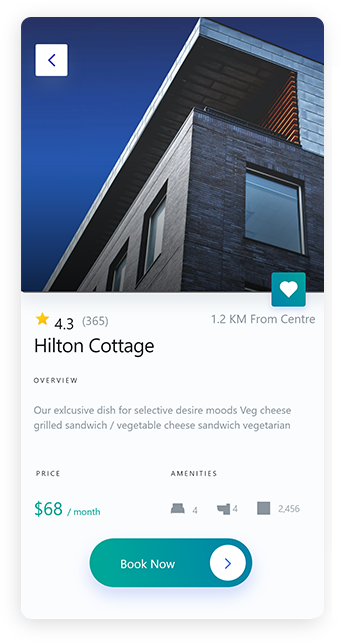The image showcases the contemporary architecture of Hilton Cottage, captured from an upward angle, emphasizing one corner of the brick building. The modern design includes numerous windows and features what appears to be a balcony extending to the roof. The background features a deep blue sky. 

Below the image is a well-organized light gray background section with various textual elements and icons. It includes a white box with a left-pointing arrow, indicating a rating of 4.3 based on 365 reviews. Additionally, it mentions that Hilton Cottage is located 1.2 kilometers from the center of town.

In the overview section, the text highlights a unique menu offering, specifically a vegetarian cheese grilled sandwich or vegetable cheese grilled sandwich, available for $68 per month. A series of amenity icons are listed, though not detailed in the caption.

Lower in the layout, there's a green gradient bar with rounded edges featuring a white circle containing an arrow pointing to the right and the text "Book Now," transitioning from light to dark green from left to right.

Overall, the image and accompanying elements create an inviting and organized presentation for potential visitors or guests.